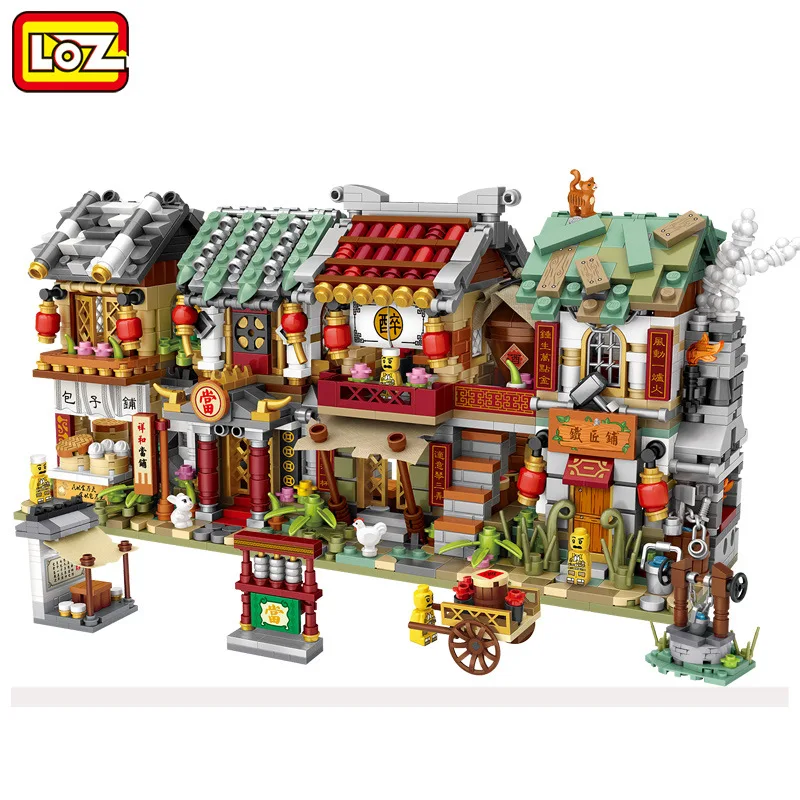This detailed image features an intricate Lego-style Asian village playset composed of eight distinct buildings arranged on two levels. Each structure showcases diverse architectural elements and vibrant colors, including green, red, yellow, gray, and white block variations. The village exudes a bustling market atmosphere filled with shops and homes adorned with Asian symbols. Notable elements include a restaurant with steam baskets and white dumplings, a shop marked by red pillars and a triangular gray roof with golden horns, and various animals like a white chicken and a rabbit.

The buildings each feature unique designs, such as roofs made from different types of blocks, like green Legos and cylinders. Several have balconies on the second floor and stairs leading up, with plants and chimneys emitting smoke adding to the lively scene. One can observe an angry-looking Lego figure outside a gray-pillared house, while another figure in a white chef's hat stands on a red, gold-tipped balcony.

In front of the buildings, the white street is bustling with activity, displaying accessories like a wooden wagon pulled by a yellow Lego figure, a well, and a tall standing item resembling an abacus. There is also a shrine-like structure used for Chinese prayers. Perched on a roof, a cat adds to the dynamic tableau. In the upper left corner, a red, yellow, and white logo within a rectangle prominently reads "LOZ," suggesting a Chinese brand akin to Lego.